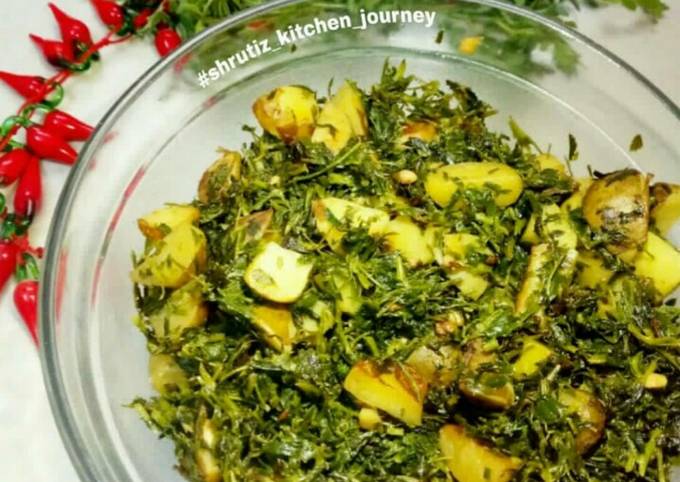This detailed color photograph captures a clear glass bowl filled with an enticing mix of chopped leafy greens, which seem to be spinach or a blend of other greens, interspersed with yellow chunks of what look like roasted potatoes. The ingredients have an oily texture, suggesting they are tossed in some type of oil. Small bits of nuts or similar small pieces are mixed throughout the dish. The bowl is surrounded by strings of what appear to be decorative red chili peppers, likely made of glass. The bowl itself is placed on a white table or background, and the photograph is taken from a top-down perspective, creating a direct view into the bowl. Written around the rim of the bowl in white font is the hashtag "Shruti's Kitchen Journey," indicating the dish's origin. In the background, small jalapenos can be seen, adding to the decor. The image beautifully showcases the vibrant colors and textures of the dish, making the food look delicious.